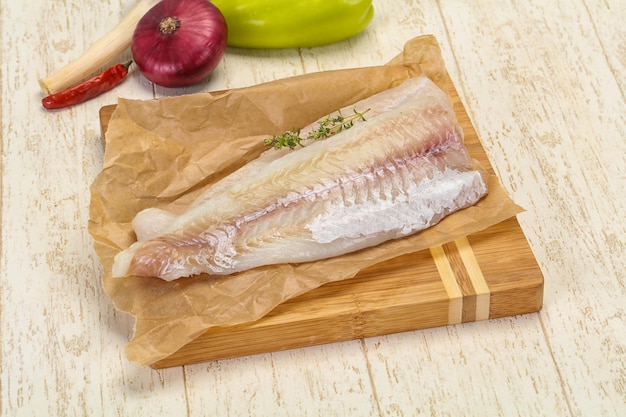In this detailed photograph, a large, white, triangular fish fillet is placed on a piece of light brown butcher paper atop a small wooden cutting board, both set on a light beige, possibly cream-colored, wooden surface. The fillet is predominantly white with hints of pink running through the center where the spines and organs were, and remnants of scales towards the bottom. A green garnish, a stem with small leaves, is thoughtfully placed on top of the fillet. Framing the fish, the top part of the image features a vibrant array of vegetables: a green bell pepper, a purple onion, and a jalapeno pepper. Additionally, a white stem is visible, contributing to the overall composition. The scene is bright, suggesting natural light amplifying the textures and fresh appeal of the ingredients displayed.